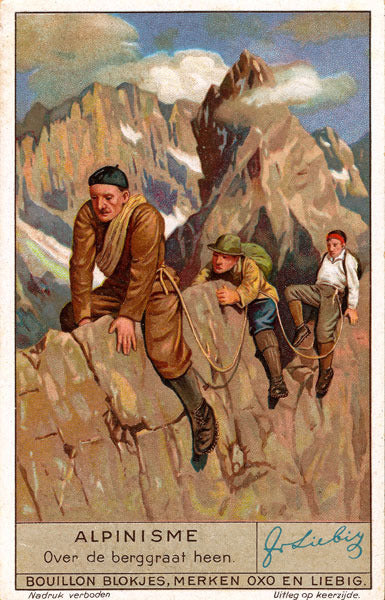This image appears to be a vintage, possibly 1920s or 1930s, hand-drawn poster of three climbers on a mountain, likely the Matterhorn given the distinctive background peaks. The climbers are connected by a rope, each in distinctive climbing attire. The lead climber, an older man in his 50s, wears a brown leather jumpsuit, brown boots, and a black hat, with a bulk of rope looping around his left shoulder and waist. The second climber, wearing a yellow jacket, blue pants, brown boots, and a green German-style hat, also carries a green backpack. The third climber at the back sports a white shirt, brown pants, dark brown low boots, red suspenders, and a red headband, alongside a backpack. All three men straddle a rugged brownish-tan ridge, with one climber sitting differently with both legs on one side. Behind them, gray, snow-capped mountains rise majestically against a blue sky with white and gray clouds. The bottom of the poster features aged parchment-like text in what seems to be German, with the prominent phrase "Alpinisme over de Bergrothin" hand-drawn in brown letters, followed by more text and a blue ink signature to the right.